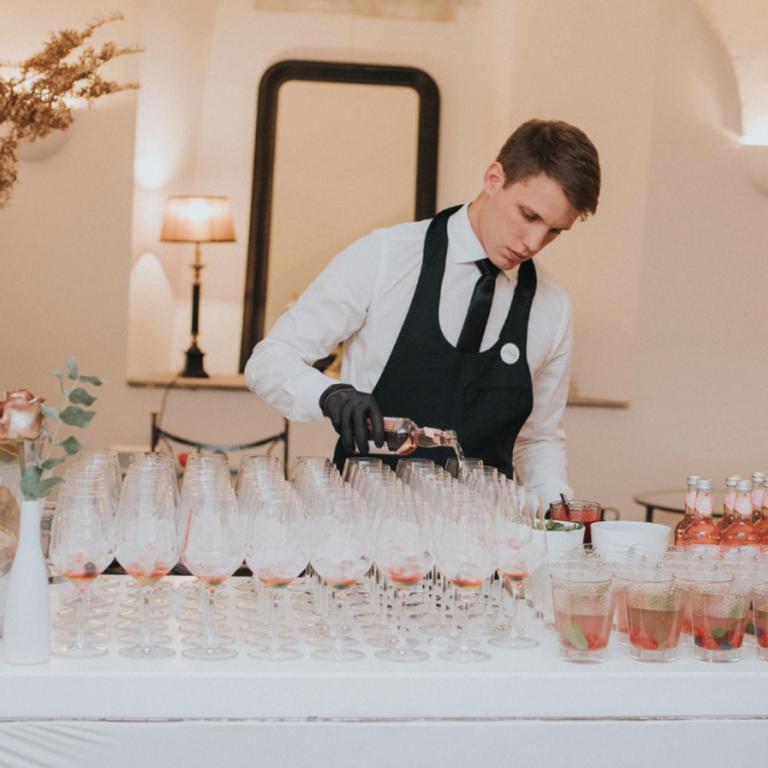The photograph captures a young white waiter meticulously pouring a pink champagne-like drink into an array of approximately 50 wine glasses, likely for a wedding or lavish event. He is dressed in a white shirt, black tie, a long black apron adorned with a round button on the left side, and black gloves. His dark hair complements his focused expression as he looks down while pouring the drinks. Around him, the table is covered with a pristine white tablecloth and also features additional cups and several bottles of the pink beverage. The elegant background reveals a well-decorated room with a brownish-beige wall, a chic mirror, a stylish lamp on a built-in table, and strategically placed lush green plants, adding to the ambiance.